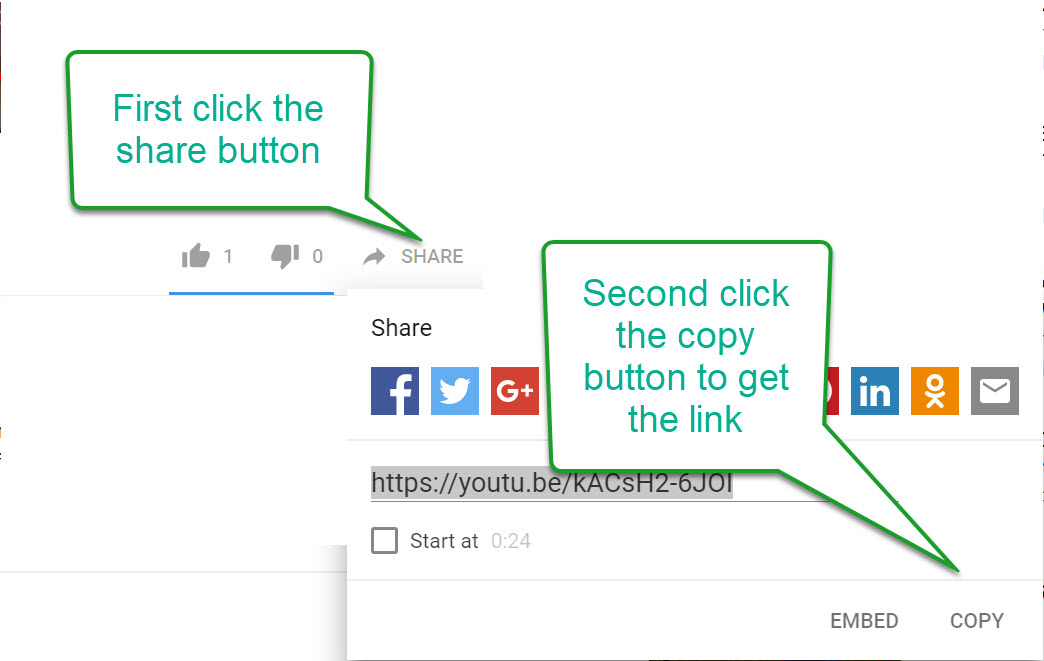This instructional illustration provides a detailed guide on how to copy and share a link, likely within the context of web design or web page functionality. The predominantly white image features multiple overlapping text boxes accompanied by instructive labels and icons.

In the upper left corner, there is a "Share" button prominently displayed alongside thumbs down and thumbs up icons. Above the "Share" button, a green bubble with an arrow points to the button, containing the directive "First click the Share button" in green text.

Overlaying this is another text box located towards the bottom right corner, labeled "Share" at the top. Within this box, icons for Facebook, Twitter, and Google are aligned horizontally. Partially obscuring these icons, a green bubble provides further instructions, specifically stating, "Second click the Copy button to get the link."

The background also includes an address bar indicating a link to YouTube. At the bottom right corner of the overlaying text box, the options "Embed" and "Copy" are displayed, reinforcing the sequential instructions.

The composition is thoughtfully arranged to guide the user through the steps of sharing a link, with clear visual cues and text for enhanced understanding.